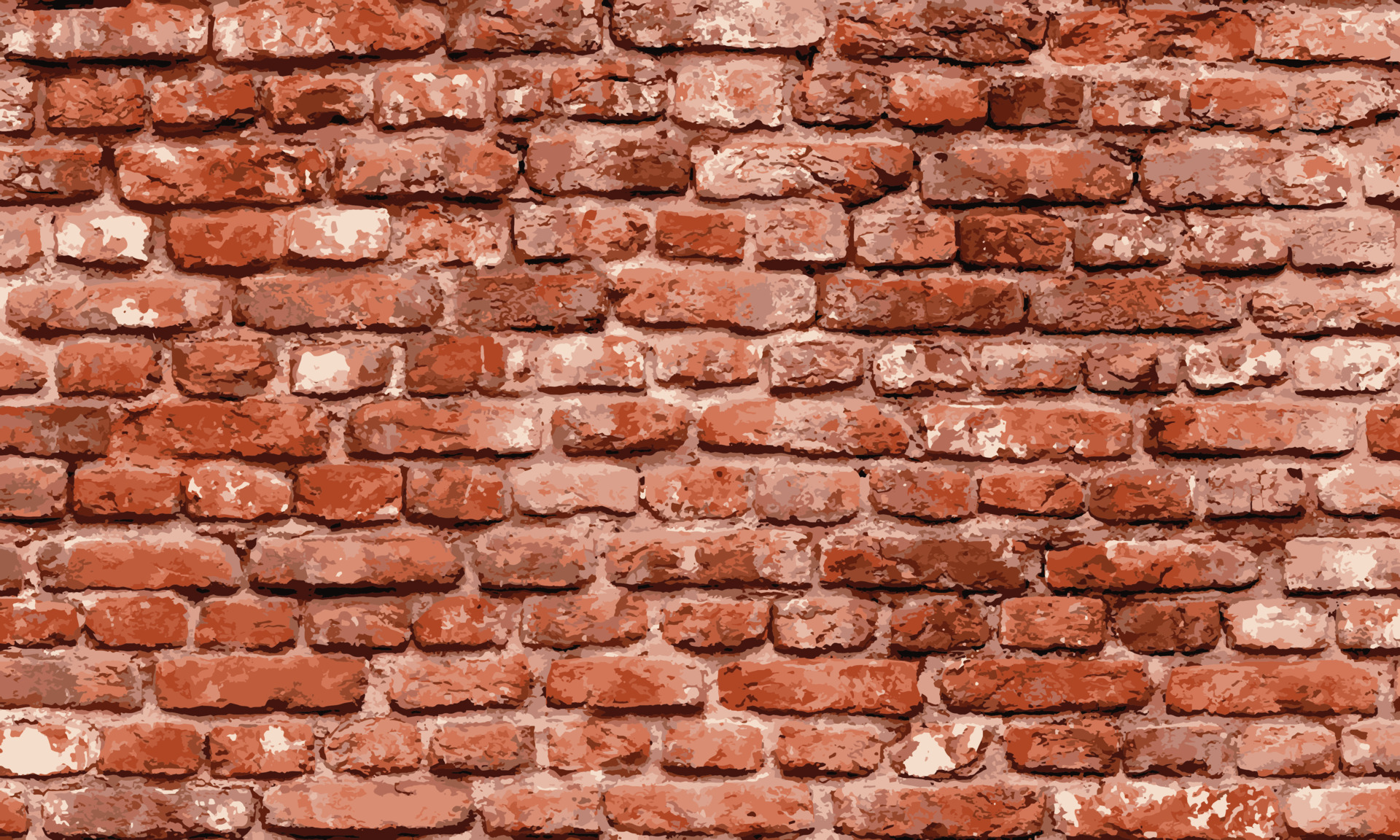This image captures a detailed view of an aged, weathered brick wall, covering the entire frame. The bricks, varying in size and shape, display an array of colors from dark and bright reds to light pinks, tans, and even spots of white, indicating significant aging and exposure. Some bricks are cracked and slightly broken, adding to the wall's character. The bricks, laid in a horizontal pattern, are bonded together by a layer of dark, muddy-colored mortar. The wall exhibits no consistent color pattern, with different shades mingling randomly. This variation in color and brick condition highlights the wall's intricate texture and historical feel.